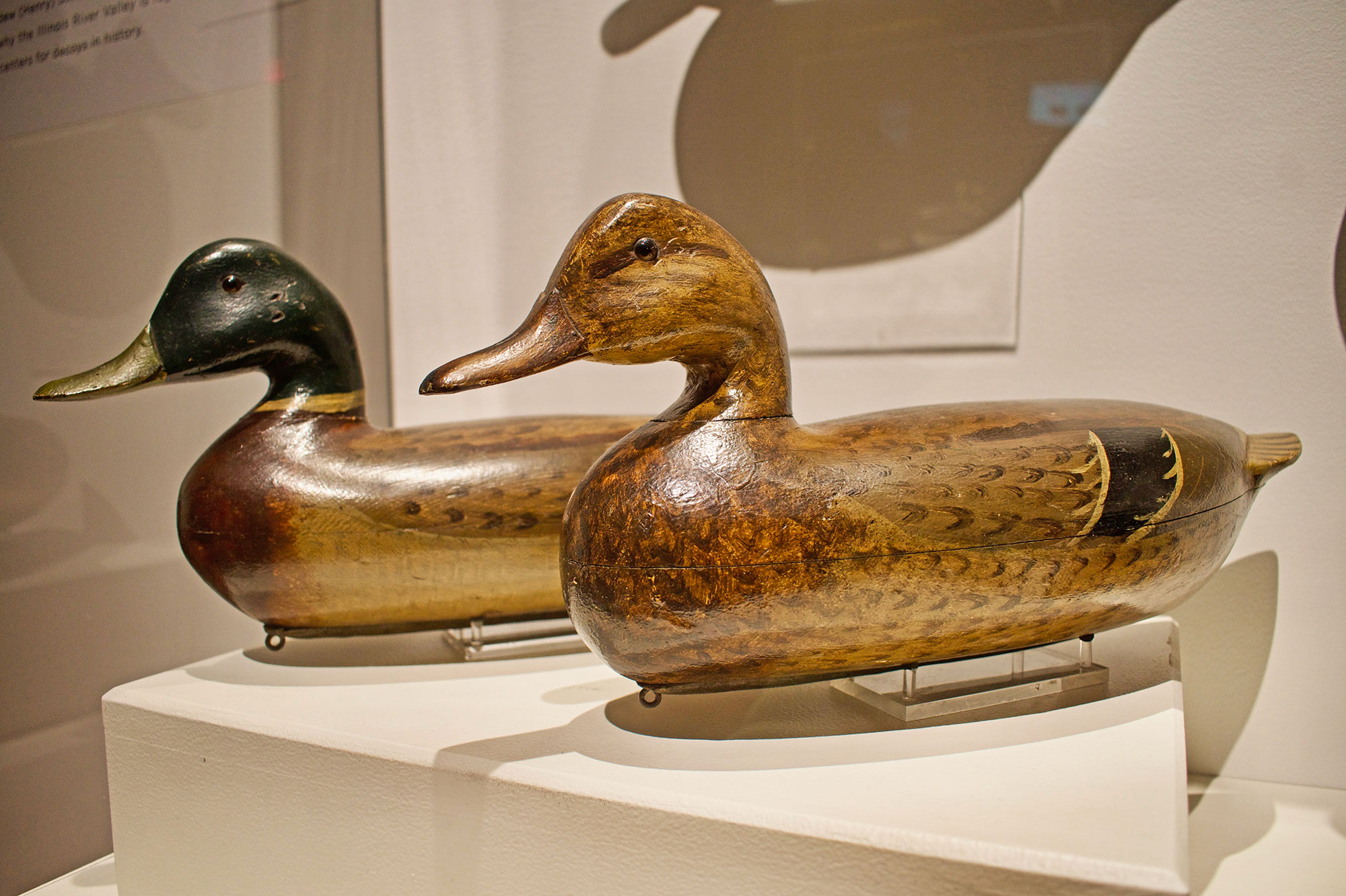The photograph captures two intricately carved wooden duck decoys, displayed prominently on acrylic stands within what appears to be a museum setting. The male and female decoys, likely mallards, rest together on a substantial beige pedestal against a similarly toned backdrop. The image is taken from a lower left angle, presenting a detailed view of the craftsmanship. The male duck, positioned on the left, features a striking green head, a distinctive stripe at the base of its neck, and a goldish bill. His brown body showcases speckles that mimic natural feather patterns. The female, foregrounded, exhibits a more subdued palette with a brown beak and facial coloring, highlighting detailed feather etching. Her wings display a broad, dark stripe bordered with gold. The overall scene includes hues of green, brown, gold, and beige, creating a naturalistic yet artistic presentation. While text is present in the upper left corner of the photograph, it remains undecipherable.